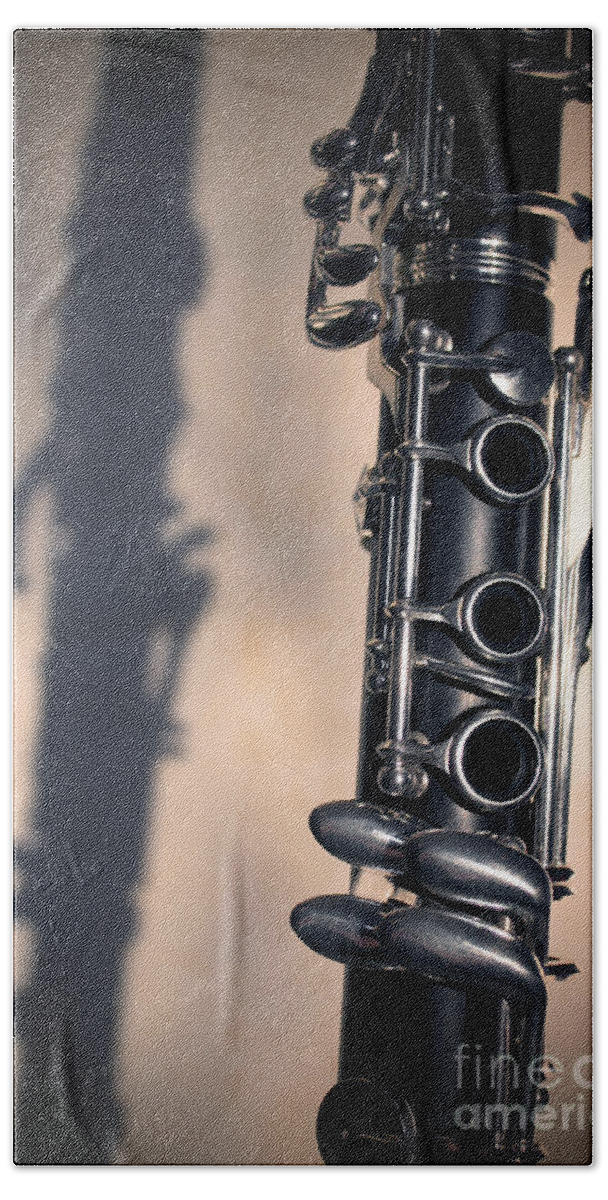The photograph is a close-up of a clarinet, captured in a slightly grainy image. The clarinet, composed of black wood and silver metal keys, is positioned upright on the right side of the frame, with only a portion visible. You can see four silver buttons on the left side along with three holes at the top, and below them, another set of four buttons arranged in two rows. The clarinet casts a distinct shadow on the left side against a pinkish-gray background. In the bottom right corner, there's a partially cut-off white watermark that reads "FINE" and "AMERI."